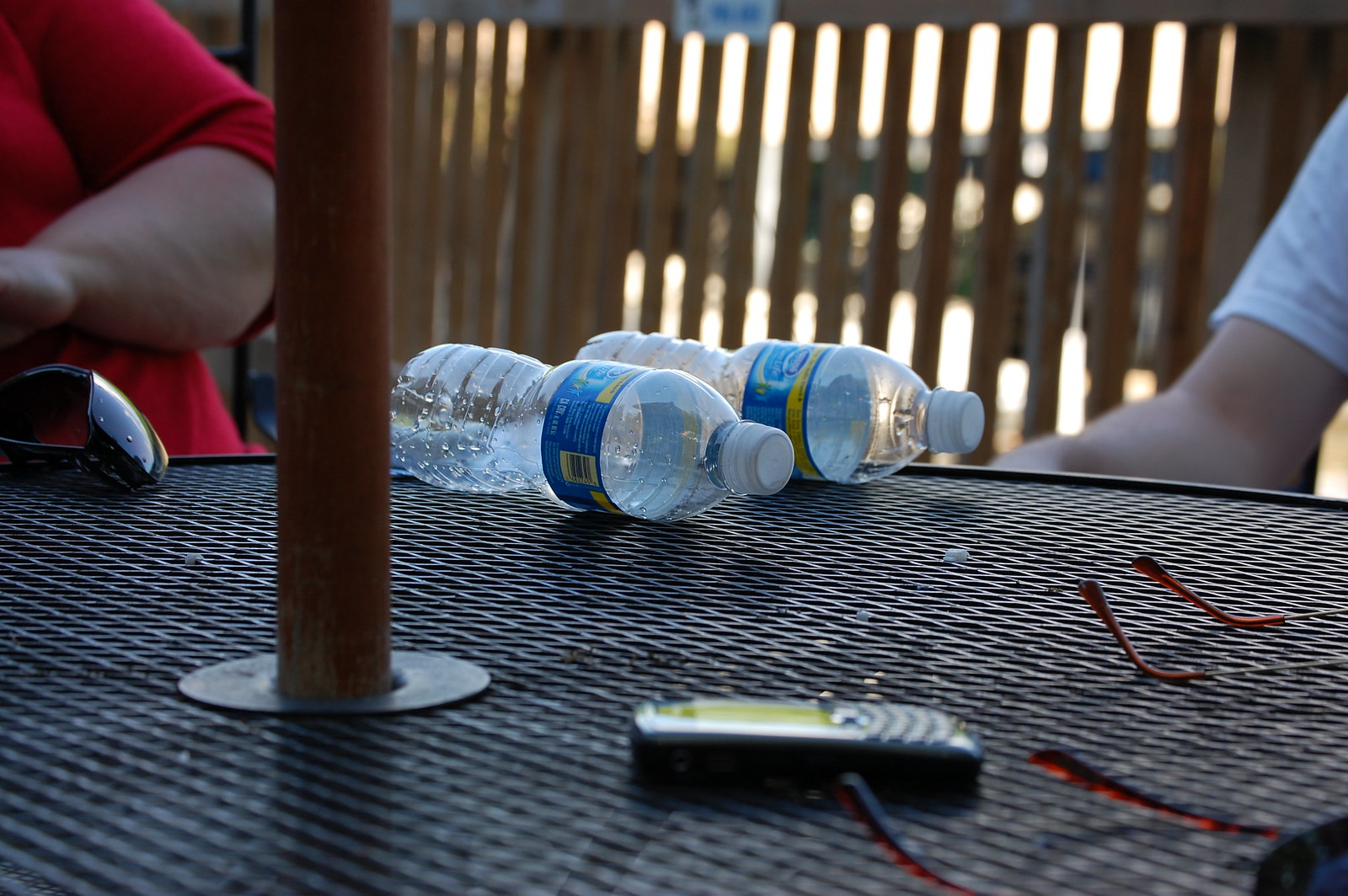This outdoor photograph captures a slightly dim-lit scene featuring a round metal picnic table with a gridded surface made of intersecting vertical and horizontal wires. Rising from the center of the table, a brown wooden umbrella pole is prominently visible. Two plastic water bottles, both tipped over on their sides and appearing empty, are positioned at the edge of the table, their caps pointing to the right. Surrounding the table, we observe two people: a woman in a red shirt on the left and another individual in a white shirt on the right, though only their arms are visible. Scattered on the table are three sets of sunglasses, a pair closest to the woman and two sets near the other person, suggesting the presence of more than two individuals. An old-style cell phone with a numeric keypad is also seen towards the front of the image. The background shows a fence and sunlight filtering through, hinting at a pleasant, sunny day, as the group enjoys their time outdoors.